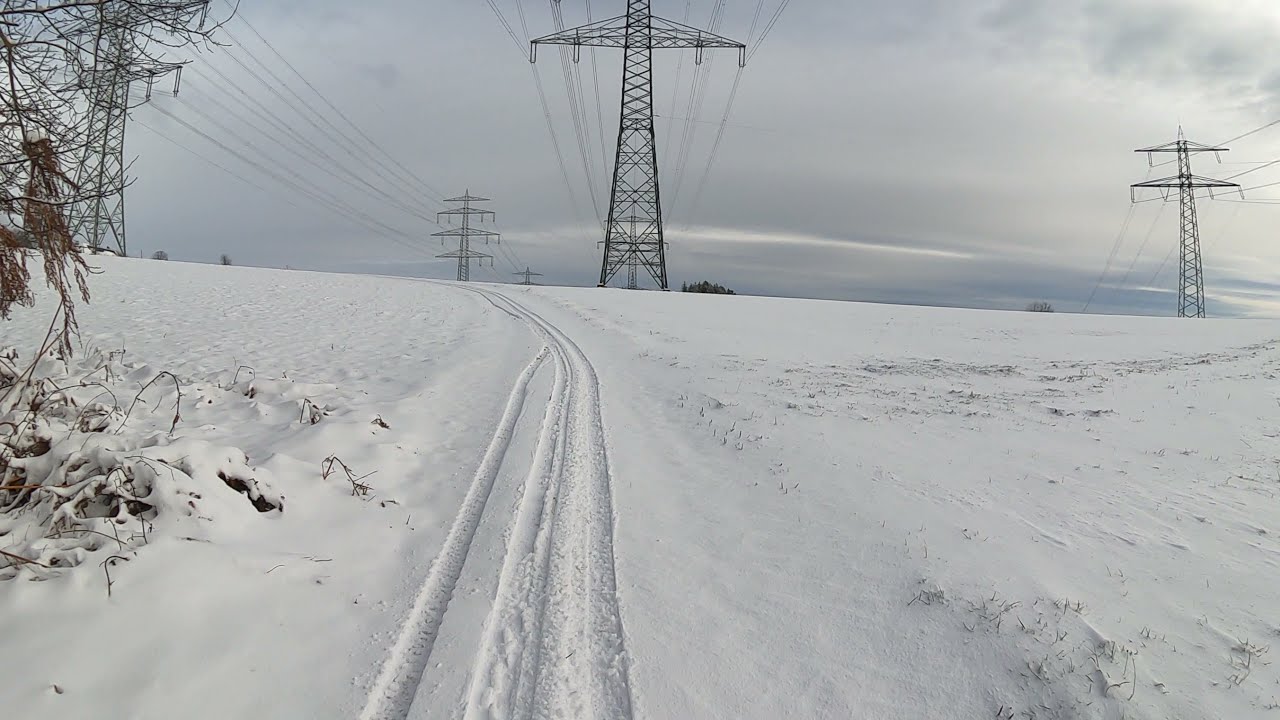The photograph, rectangular in shape, captures a winter landscape taken from ground level, looking up a snow-covered hill. The sky above is a blend of gray and blue, heavily clouded, typical of an overcast day. Dominating the scene, there are four towering power line structures; one stands much closer to the foreground, drawing immediate attention, while the others recede into the distance. The ground, blanketed in fresh, white snow, features distinct, narrow tracks likely made by a snowmobile carving its path uphill. To the left of the image, just ahead of the snowmobile tracks, the edge of some barren shrubbery is visible, its lifeless branches reaching out. Beneath this foliage, patches of tall grass and weeds protrude through the snow, indicating a layer thin enough to let nature break its surface. There are no people present, emphasizing the serene and somewhat desolate wintry environment.